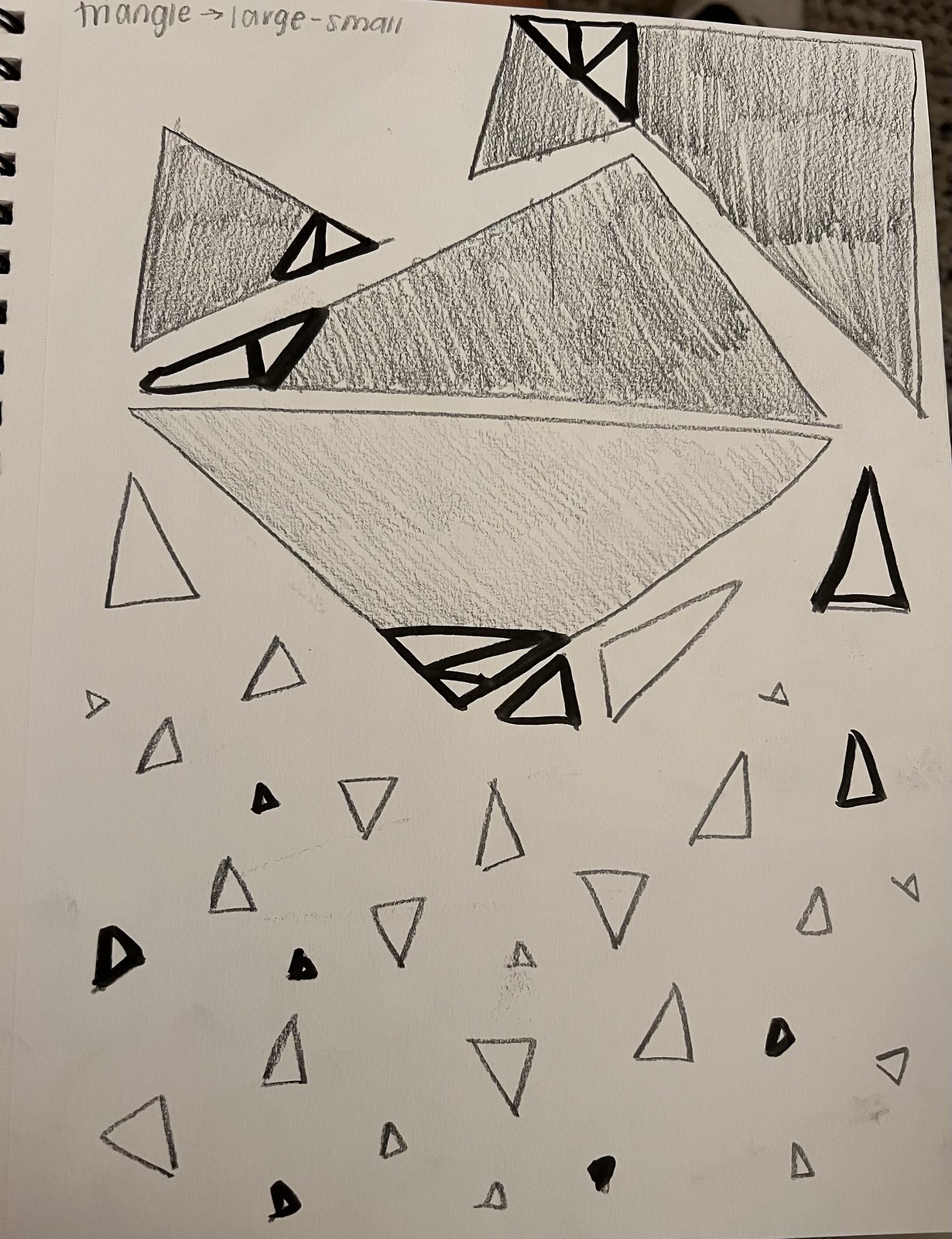A detailed pencil and marker sketch on plain white paper within a spiral-bound notebook. At the top of the page, the words "Triangle and Arrow - Large to Small" are inscribed. The drawing features an array of triangles, initially drawn with a pencil or possibly black crayon. Several of these triangles have been traced over with a black magic marker. Some triangles are further subdivided into smaller triangles, with all subdivisions emphasized using the black marker. The overall effect showcases the evolution of simple geometric shapes into more complex structures, highlighted by the stark contrast between the softer pencil lines and the bold marker strokes.